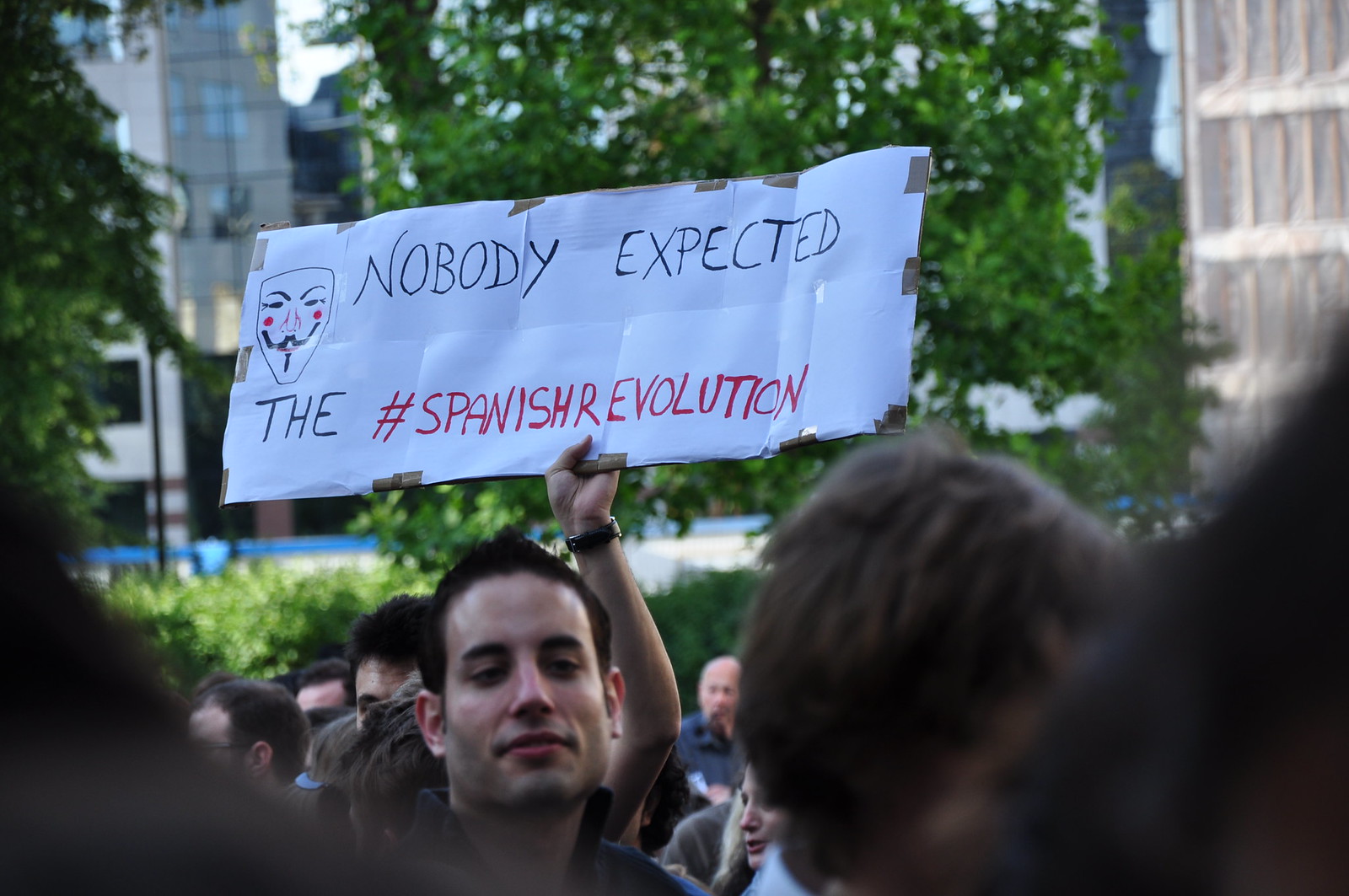The image depicts a group of people gathered at what appears to be a protest event, set against an urban backdrop with modern skyscrapers. Despite the city setting, the scene also features greenery with trees, bushes, and a field of grass in the foreground, which suggests the gathering might be taking place in a park or boulevard. Centrally featured in the crowd, someone is holding a large white sign composed of multiple 8x11 sheets of printer paper taped together on a solid backing. The sign prominently displays a hand-drawn mask with a mustache, eyebrows, red rosy cheeks, and a semi-smiling mouth. Handwritten text in black marker at the top of the sign reads "Nobody expected" and at the bottom, in black, "the" followed by "hashtag Spanish Revolution" in red. The men in the group appear partially visible, with one particularly noticeable young man who is not holding the sign but standing below it, looking down. The photograph, seemingly taken through the branches of a tree, creates a semi-framed effect with some blurry brown edges.